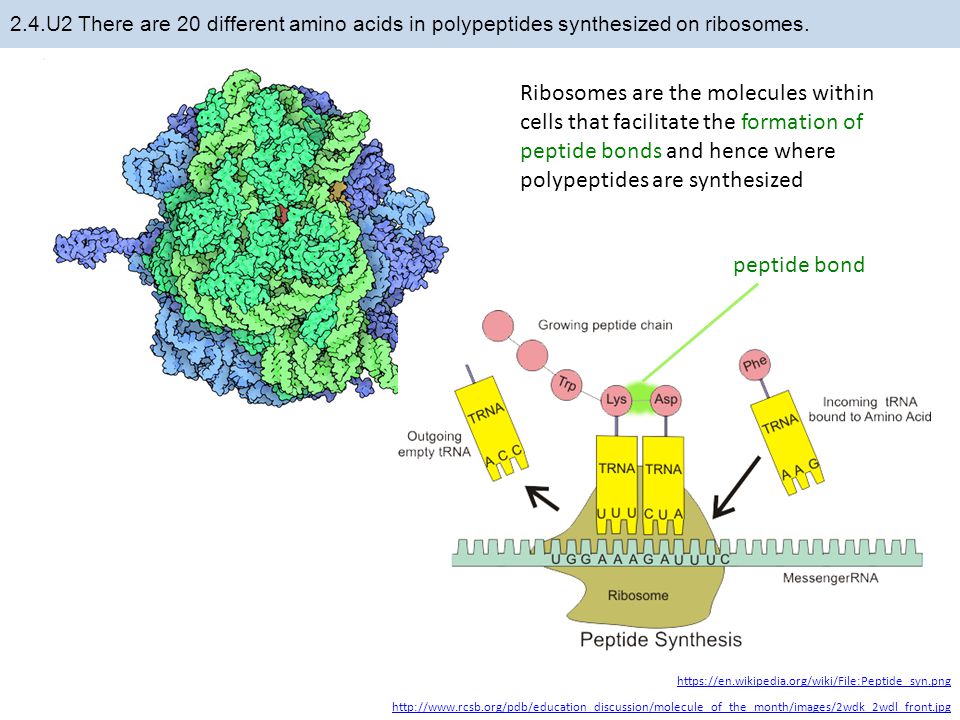The slide is an informational presentation about peptide synthesis, focusing on the role of ribosomes. The background is predominantly white with various black lines of text and graphics illustrating the concepts. At the very top, there is a light blue banner stretching from left to right, featuring black text that reads "2.4.U2." Below the banner, there is a paragraph stating, "There are 20 different amino acids in polypeptides synthesized on ribosomes. Ribosomes are the molecules within cells that facilitate the formation of peptide bonds and hence where polypeptides are synthesized." On the left-hand side of the slide, there is an intricate, colorful illustration composed of blue, purple, lime green, and dark green lines tangled together, likely representing the complex structure of ribosomes or a related cellular process. Below this, there is a detailed diagram showing a growing peptide chain and peptide bond formation, as well as elements of DNA and RNA connecting, visually explaining the steps of peptide synthesis. The slide is part of a comprehensive medical or educational presentation, designed to give a thorough understanding of ribosomes' role in peptide bond formation and polypeptide synthesis.